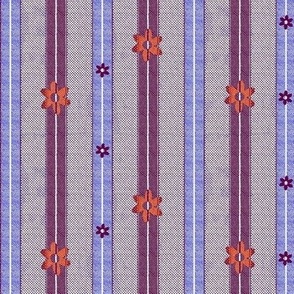The image is a detailed photograph of a section of striped fabric, possibly used for upholstery or drapery, featuring a vintage design. The fabric presents alternating vertical stripes in blue, lavender, purple, and gray shades. Each stripe is adorned with unique floral patterns and thin white lines running down the center. The purple stripes showcase orange six-petaled flowers that are precisely aligned along the white lines. On the blue stripes, tiny purple flowers with white centers appear, with one stripe having three flowers and another having four. The gray background fabric is visible between the colored stripes, adding to the intricate and old-fashioned aesthetic.